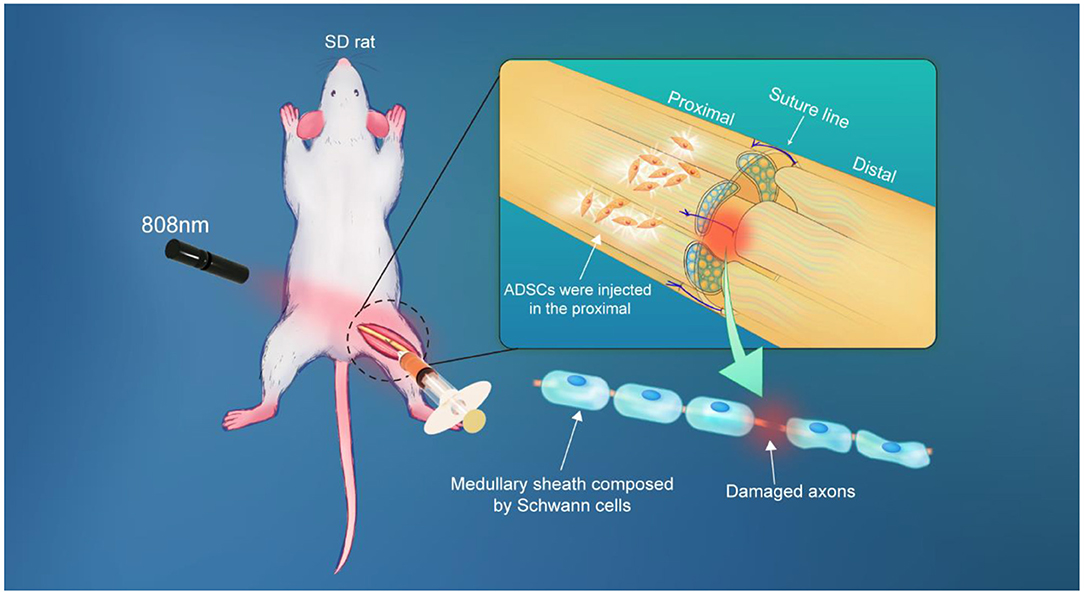The image depicts a detailed medical diagram with a dark to medium blue background, focusing on a rat labeled "SD rat" drawn in white. The rat features pink paws, ears, nose, and a long pink tail, with its four limbs splayed out. To the left of the rat, there is a black tool marked "808 NM" with an emitting pink (or red) light directed at the rat's left rear thigh, highlighting an opened section of skin where a needle is being inserted.

Above the rat, the text "SD rat" is displayed in white, indicating the subject's species. The needle insertion point is circled in black, showing an incision area. A detailed inset magnifies this site, revealing a complex view of a yellow tube-like structure labeled with "proximal" and "distal." The proximal end notes the injection site of ADSCs (Adipose-Derived Stem Cells), emphasized by arrows pointing to tiny oblong orange objects with white radiating lines. 

Above the yellow tube, text indicates "suture line," marking a central red incision point and showing small green and yellow squiggles in a cross-section. Additionally, another arrow points to blue oblong shapes identified as "medullary sheath composed of Schwann cells." A further highlighted section marked by a red blur shows disrupted parts labeled "damaged axons," completing the depiction of this intricate medical procedure and its anatomical focus.